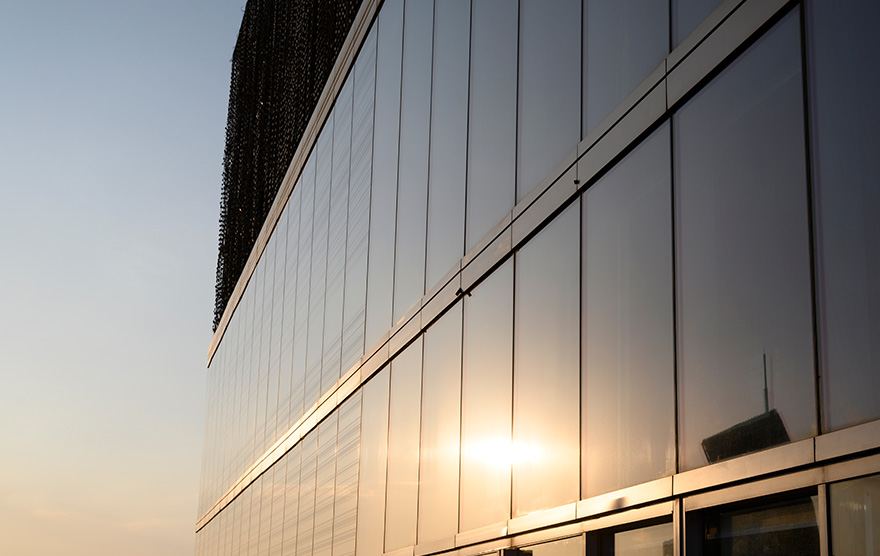This photograph captures a striking image of a multi-story, commercial office building made predominantly of reflective glass panels. The building's facade features two to three visible rows of vertical, floor-to-ceiling, rectangular panes, with horizontal lines bisecting them. The top section of the building shows a black structural element, possibly railings or chains. The photo appears to be taken during sunset, as the sky to the left transitions from dark blue to light blue and then to a pinkish-orange hue, which reflects beautifully off the glass panels, giving them a pinkish glow. Below, near the bottom of the image, there's a glimpse of what seems to be a sliding door. The sunlight is intensely bright and reflects off about six of the visible glass panes, highlighting their polished surface.